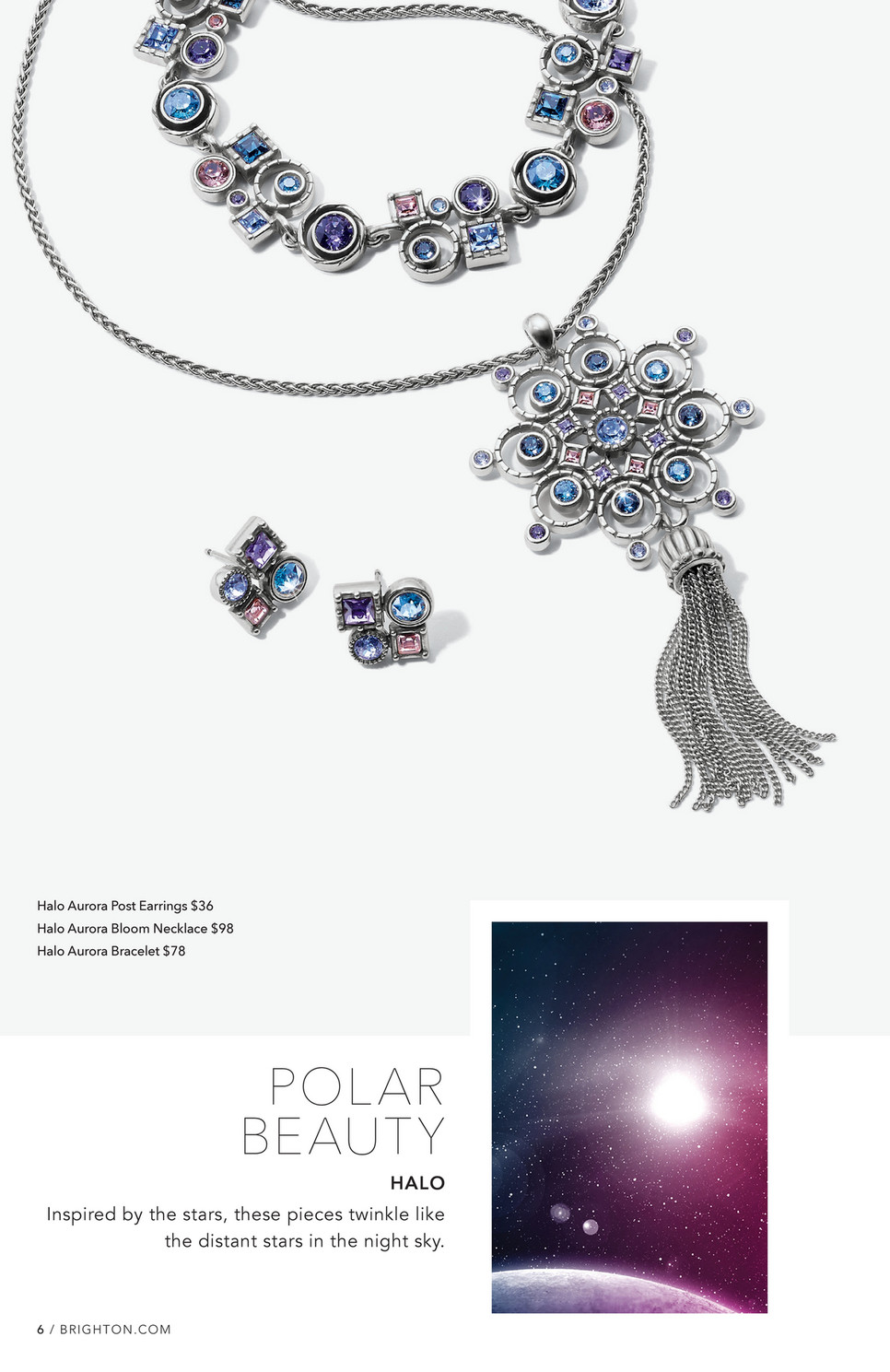This promotional poster features a vertically oriented rectangular design with a light gray background. The upper portion showcases an array of silver jewelry, including a large, ornate necklace with turquoise and various gemstones in shades of blue, purple, and pink, designed with circular, triangular, and square elements, and featuring a silver chain tassel. Complementary pieces consist of a pair of earrings featuring a similar multicolored gem arrangement and a potential bracelet or decorative necklace. Accompanying the jewelry in black text are the descriptions "Halo Aurora Post Earrings, $36," "Halo Aurora Bloom Necklace, $98," and "Halo Aurora Bracelet, $78."

The bottom section displays an evocative photograph with hues of purple and blue, depicting a cosmic scene with a shining star above a planet. Large white text labels this section "Polar Beauty," with smaller text reading "Halo," accompanied by the phrase "Inspired by the stars. These pieces twinkle like the distant stars in the midnight sky."